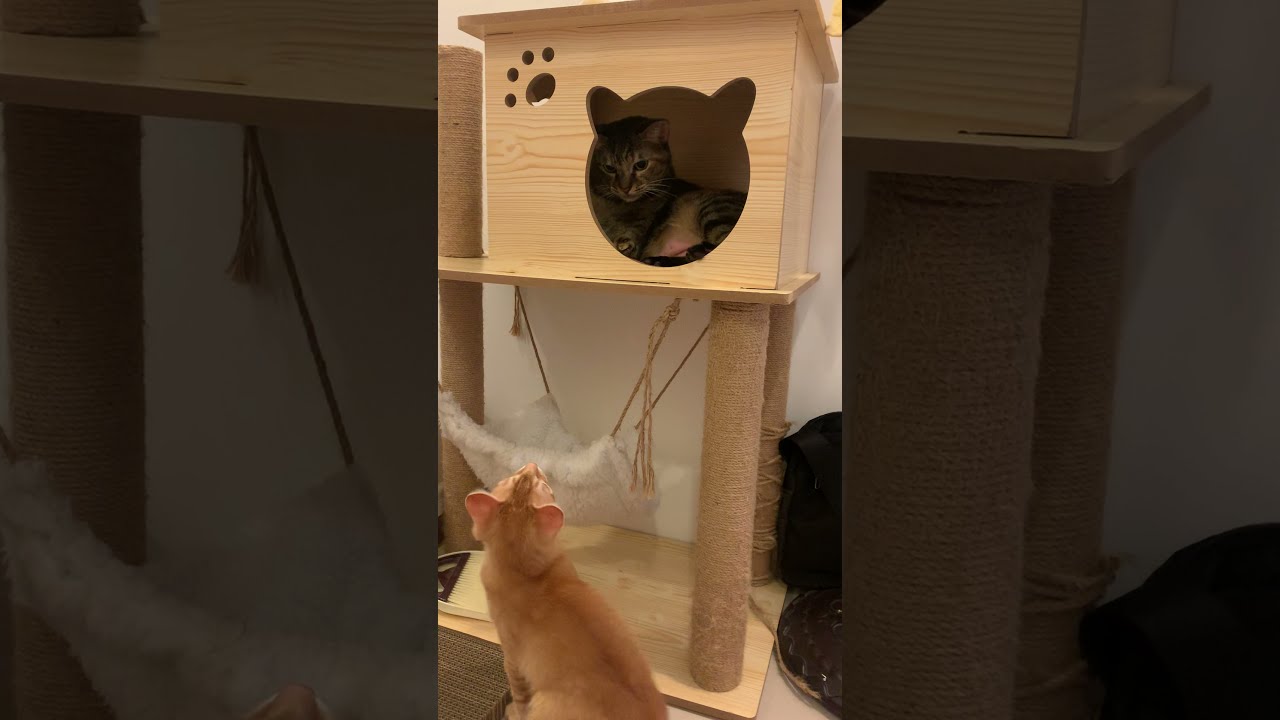The image consists of three panels: a central photo flanked by two detailed blow-ups of the photo's sides. The central panel showcases a cat play structure with two stories. The left and right panels, which are underexposed and dark, zoom in on each side of the play structure. On the second story of the play structure, there is a small enclosure with an entrance shaped like a cat's head, complete with ears—a gray tabby cat perches inside, resting and peering down. The structure is supported by four posts wrapped in jute rope, which looks scratchy. Below, a white, furry cat hammock is suspended between the posts. On the ground floor, a light brown tabby cat gazes upwards toward the enclosure, engaging in a silent exchange with the gray tabby above. The setting appears to be an indoor room, possibly a den, indicated by the presence of a work table in the background.